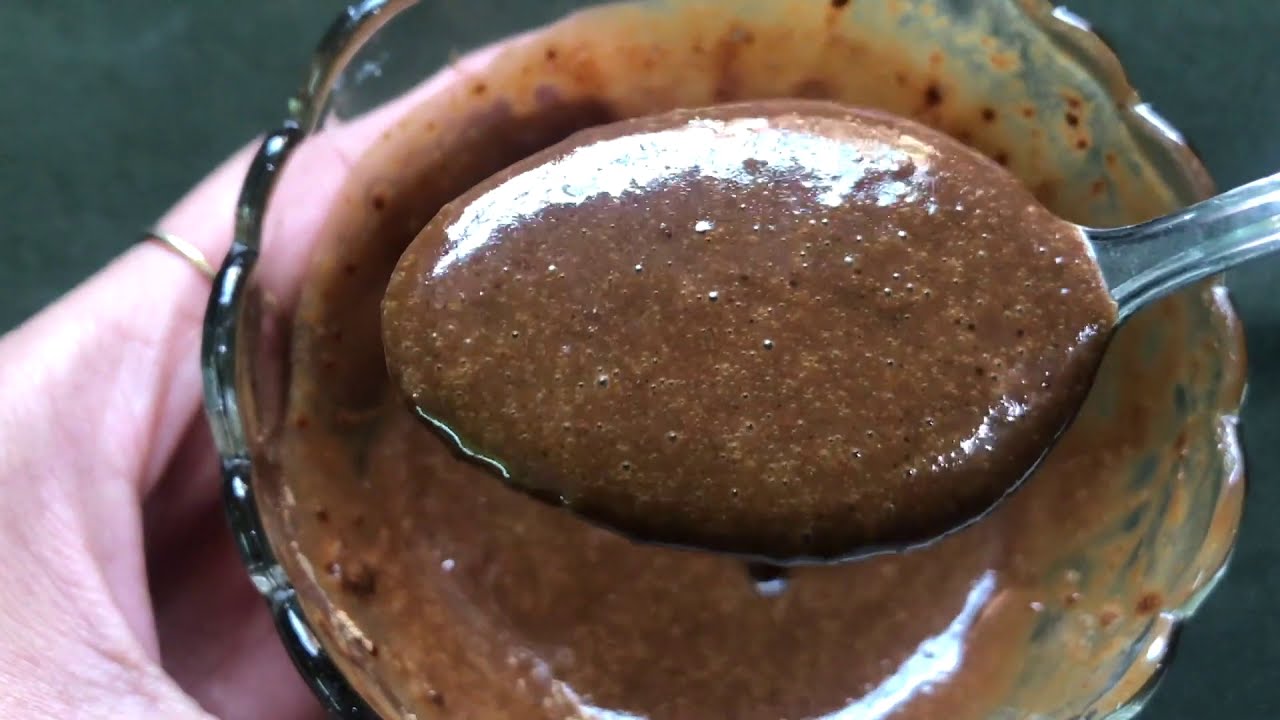This horizontal rectangular image showcases a close-up of a person's hand, adorned with a ring on their index finger, holding a round glass bowl filled with a dense, dark chocolate-brown liquid. The hand is partially blurred in the lower left-hand corner. The bowl, possibly an ice cream sundae dish, is the prominent feature and occupies the center of the image. A glistening silver spoon extends from the right side, its handle reaching out of the frame, with its bowl section containing the same chocolate-brown substance, which features tiny bubbles and darker specks. The edges of the glass container show smears of the liquid, adding to the texture. The background of the image consists of a darker gray hue in the upper left, upper right, and lower right corners, creating a stark contrast with the rich, inviting tones of the chocolate inside the bowl.